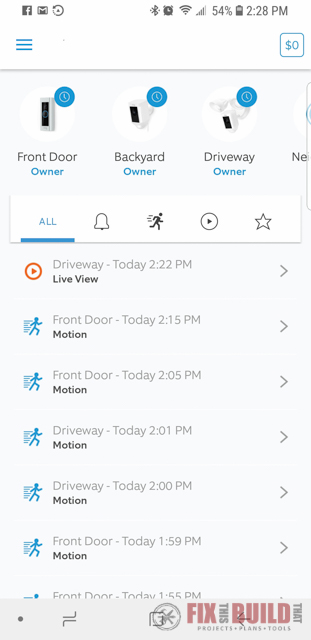A vertical image depicts a user interface of a security camera application accessed via a smart device. At the top, there are various icons including social media symbols on the left, and Bluetooth, Wi-Fi, clock (showing 2:28 p.m.), signal strength, battery life (54%), and more options (represented by three horizontal blue lines) on the right. Adjacent to these icons on the right is a blue square with a "$0".

The main section of the image shows different security camera feeds labeled "Front Door Owner," "Back Door Owner," and "Driveway Owner." An options menu is prominently displayed with selectable icons for "All" (currently highlighted in blue), an alarm bell, a running person, a play button, and a star.

Below the camera feeds, there is a history log of recent activities. Each entry includes a timestamp and a brief description. For example, at 2:22 p.m., the log indicates a live view from the driveway, marked with a red triangle; at 2:15 p.m., there's a motion detected at the front door; followed by various other motion detections at the front door and driveway at 2:05 p.m., 2:01 p.m., 2:00 p.m., and 1:59 p.m. The log entry for 1:25 p.m. is partially cut off. At the bottom of the interface, there is an icon suggesting the user can access settings or make adjustments.